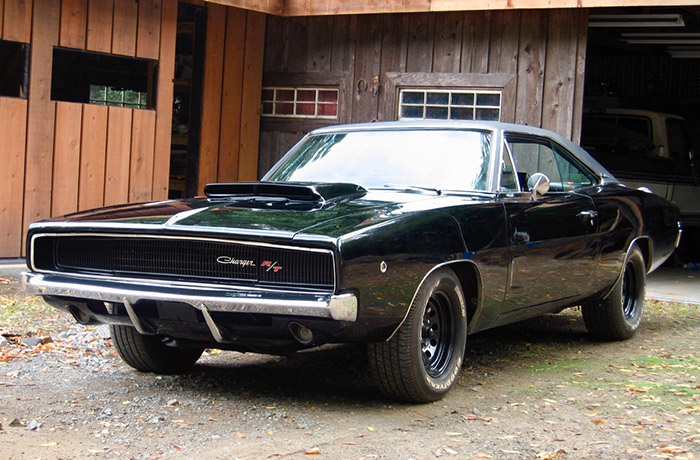The image features a vintage Dodge Charger, reminiscent of classic TV shows such as Starsky and Hutch. The car is a striking emerald green, with a sleek two-door design and a distinctive long rectangular grille bearing the name "Charger" in cursive script alongside an "R/T" symbol. The "R" and "T" letters are highlighted in red. It appears to have a convertible top, and the front windows are rolled down, revealing a sunlit windshield. The Charger is parked in a dirt and gravel driveway, surrounded by fallen leaves, in front of a rustic wooden garage with intersecting sliding doors of contrasting dark and light wood. Eye-level windows and a horseshoe symbol adorn the garage doors, adding a farm-like ambiance to the scene. Behind the Charger, inside the garage, an old truck with green and white stripes is visible, further contributing to the nostalgic, rural setting.